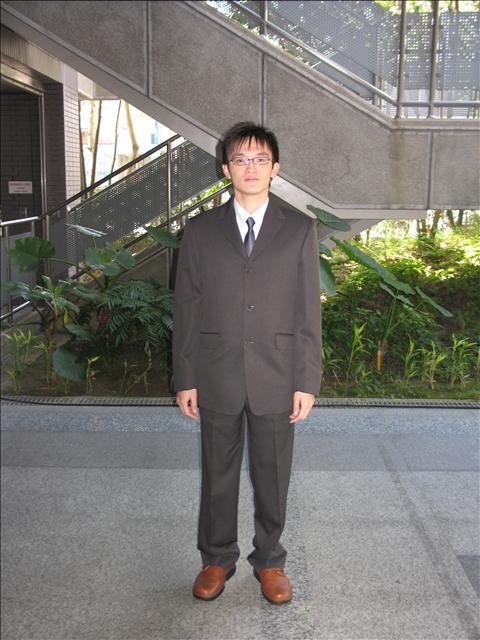The photograph showcases a young Asian man standing outdoors on a walkway comprised of large square tiles speckled with gray and black. He is gazing forward with his arms resting at his sides, exuding a composed demeanor. The man sports black-rimmed glasses and has black hair styled slightly downward.

He is dressed formally in a black dress coat buttoned up with three black buttons, revealing a white collared shirt underneath and a grayish-blue tie. His outfit is completed with black dress pants and light brown leather dress shoes featuring black soles. 

Behind him, a landscaped area with lush green grass separates him from a distinctive staircase with gray stone walls and metallic handrails. The staircase, which initially ascends to the right, then moves forward and further ascends to the left, creates a notable backdrop, along with a thin, bright window further back. Additionally, a dark door is visible on the left side of the image, complementing the overall outdoor setting.